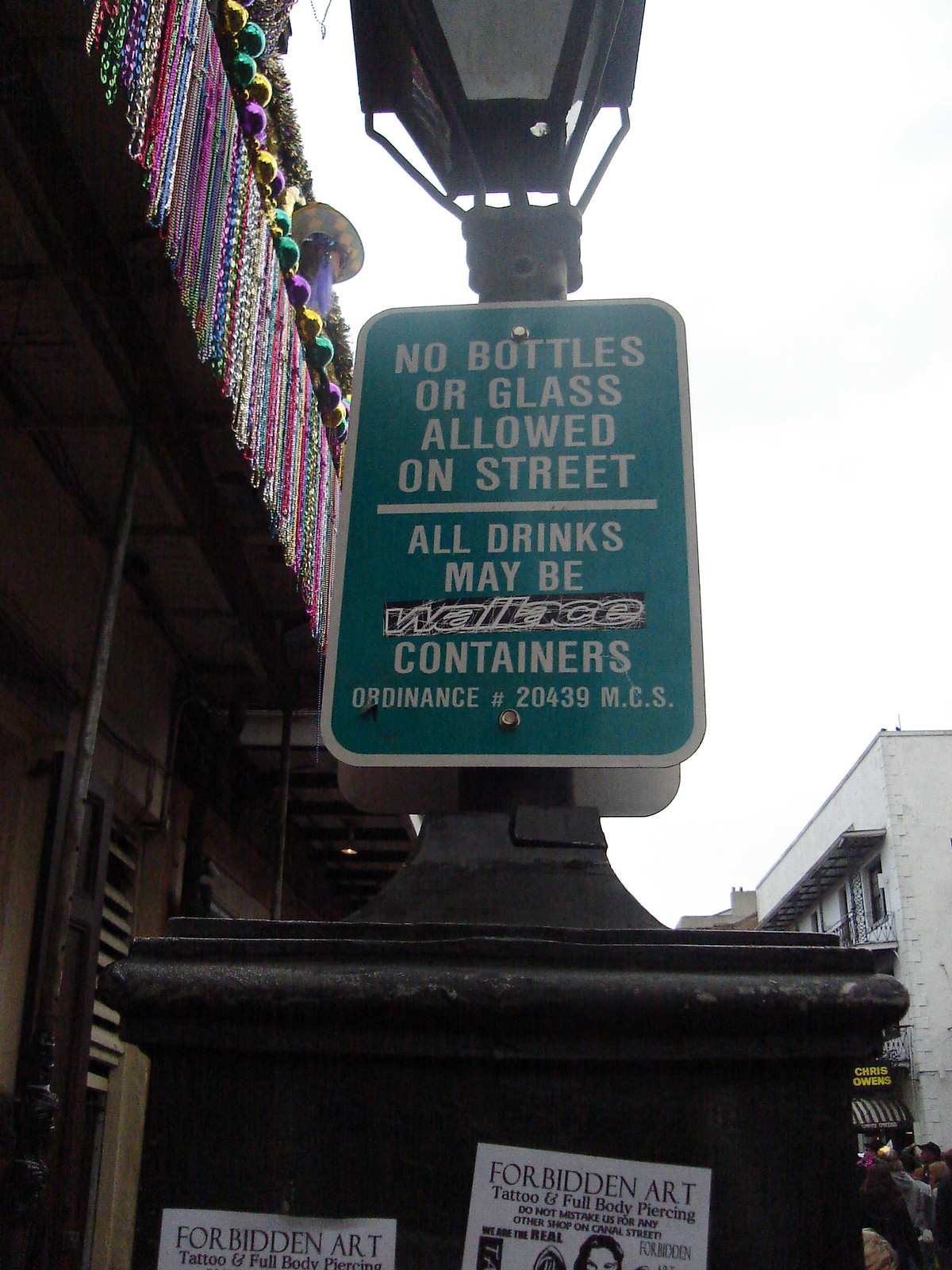The image is a tall rectangular photo centered around a street sign mounted on a black metal lamppost. The upper portion of the lamp is cut off at the top of the image. The green sign with a thick white border is positioned in the middle of the post and reads in white capital letters, "NO BOTTLES OR GLASS ALLOWED ON STREET." Below this, separated by a horizontal line, it continues, "ALL DRINKS MAY BE CONTAINERS," obscured by a black italicized sticker reading "Wallace." The bottom of the sign displays "ORDINANCE NUMBER 20439 MCS."

In addition to the sign, the background features various buildings and a bustling city atmosphere. On the left side, there’s a two-story building adorned with multi-colored, Mardi Gras style decorative ribbons and beads hanging from the second level. To the right, there are more buildings and a crowd of people visible. The overall scene suggests a downtown area during daylight.

Conclusively, the photo captures the vibrancy of an outdoor city setting with detailed elements of urban decor and public regulations peppered with a hint of local vandalism.